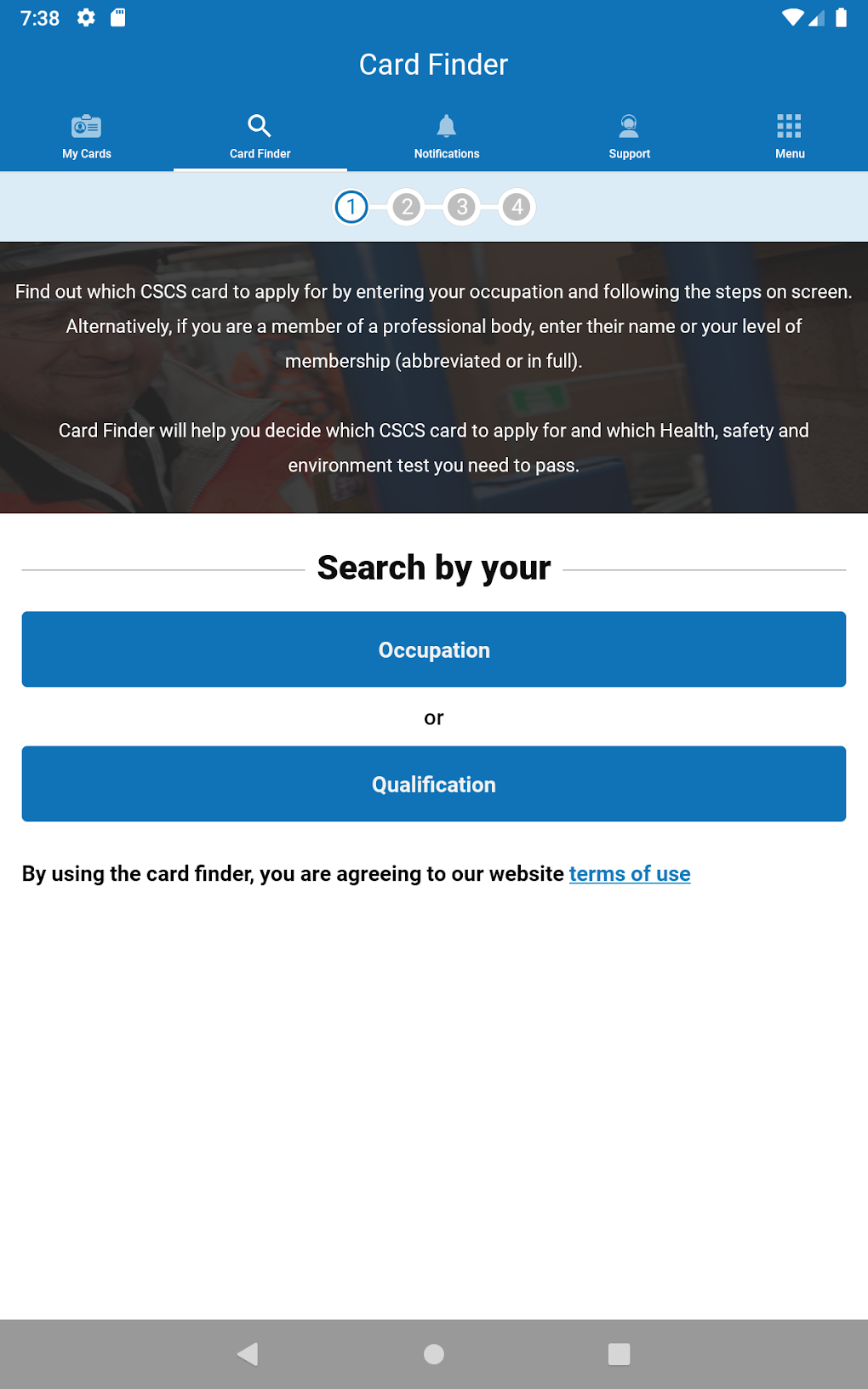The image displays a smartphone screen showcasing a webpage with a blue header. At the very top, the time is shown as 7:08, along with icons for settings, SD card, Wi-Fi signal, and battery status in the top right corner. Centered beneath these icons is the text "Card Finder." Below this header is a navigation bar with tabs labeled "My Card," "Card Finder," "Notifications," "Support," and "Menu," with "Card Finder" highlighted.

The main content area is organized into a series of four steps, with Step 1 currently highlighted in blue. The step's instructional text appears in white against a dark background and reads: "Find out which CSCS card to apply for by entering your occupation and the following steps on the screen. Alternatively, if you are a member of a professional body, enter their name or your level of membership, abbreviated or in full. Card Finder will help you decide which CSCS card to apply for and which health and safety and environmental test you need to pass."

Below this instruction, the prompt "Search by" is displayed, followed by two blue buttons labeled "Occupation" and "Qualification" with white text. At the bottom of the screen, there is a note in black text stating, "By using the Card Finder, you are agreeing to our website terms of use," with "terms of use" highlighted in blue.